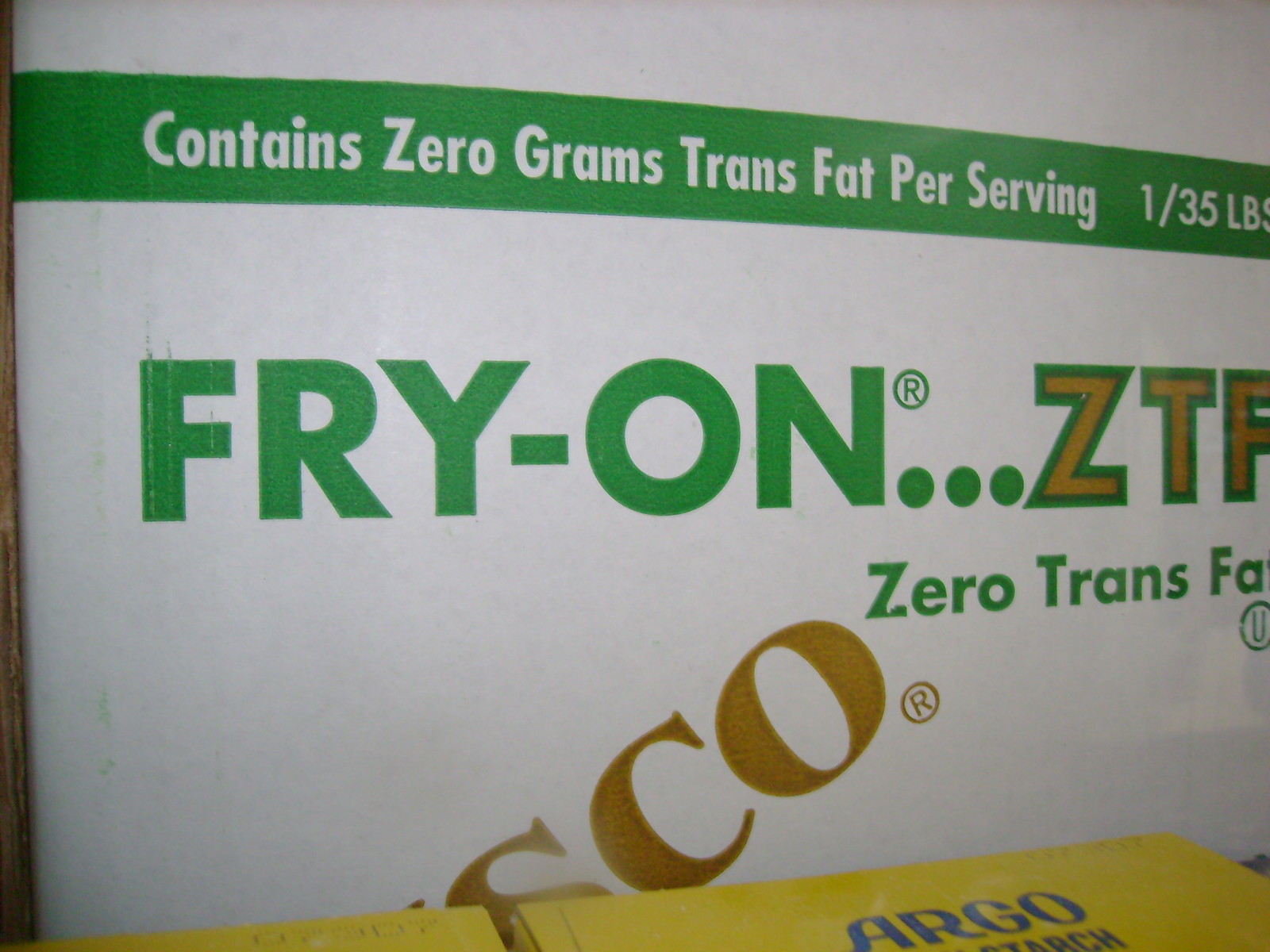This photograph showcases a white product packaging box with detailed branding and nutritional information. A prominent green bar spans the top of the box, highlighting that the product contains zero grams of trans fat per serving and weighs 1.35 pounds. Central to the design, the box features the phrase "Fry On..." in green text. Below this, the acronym "ZTF" is written in bold brown letters with a green outline, with "Zero Trans Fat" displayed in smaller green text beneath it. Additionally, a yellow box appears at the bottom right corner, containing the word "Orgo" in bold blue text.